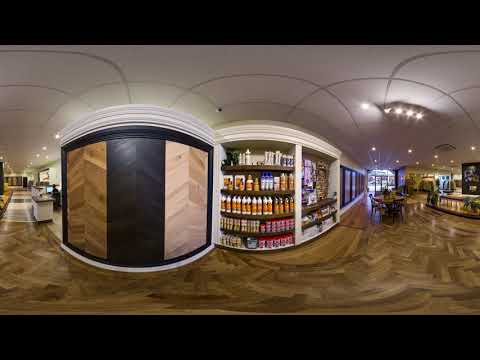This panoramic, fisheye-view photograph captures a sophisticated, upscale store interior, possibly a luxury spa or beauty salon. The image reveals a polished, zigzag-patterned hardwood floor varying in shades of brown that accentuates the lavish atmosphere. The ceiling is tall, arched, and pristine white, adorned with intricate designs and bright, recessed lighting fixtures. Centrally located, an aisle with five rows of neatly arranged shelves displays an array of products, likely shampoos, body care items, or beverages. The shelves, designed with a combination of white and brown tones, extend towards the background, emphasizing the store's spaciousness. 

On the left of the image, a service station—potentially for hair cutting or facial massage—features a parquet wood display with panels in lighter brown, black, and light green. A person stands at this station, adding a dynamic element to the space. The left foreground also highlights what resembles a tanning or spa booth, further underscoring the store's luxury appeal.

Towards the middle, a table accompanied by chairs provides a resting or consultation area. Near the right-hand side of the photograph, a well-lit reception desk is positioned close to a doorway leading to the store from the street. This comprehensive view, characterized by the fisheye lens's unnatural curves, encapsulates the elegant and polished ambiance of this high-end establishment.